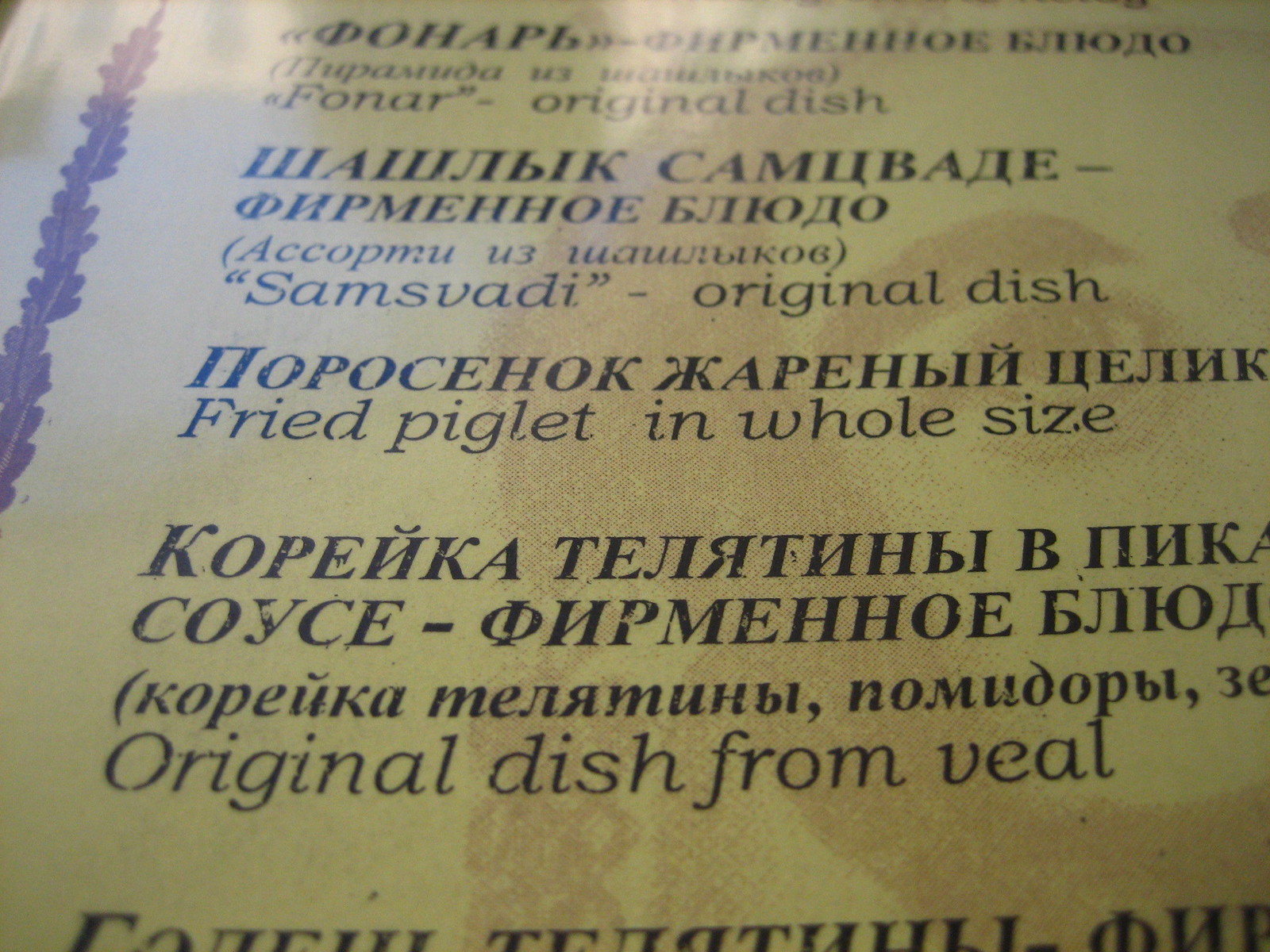A close-up image of a Russian restaurant's menu, printed on cream-colored paper. The menu features prominent headings in bold Russian text, with English translations provided. The title "Phonar" appears at the top as an original dish, accompanied by a brief description in Russian, which includes a parenthetical explanatory phrase that remains untranslated. A distinctive red banner, resembling a stem or branch with small growths, runs vertically along the side of the menu, serving as a decorative element. The menu items include a variety of traditional dishes, with entries such as "Sam's Vadi," described as an original dish, and "Fried Piglet in Whole Size," along with "Original Dish from Veal." The menu offers detailed explanations for each dish in both Russian and English, providing a comprehensive guide for diners.